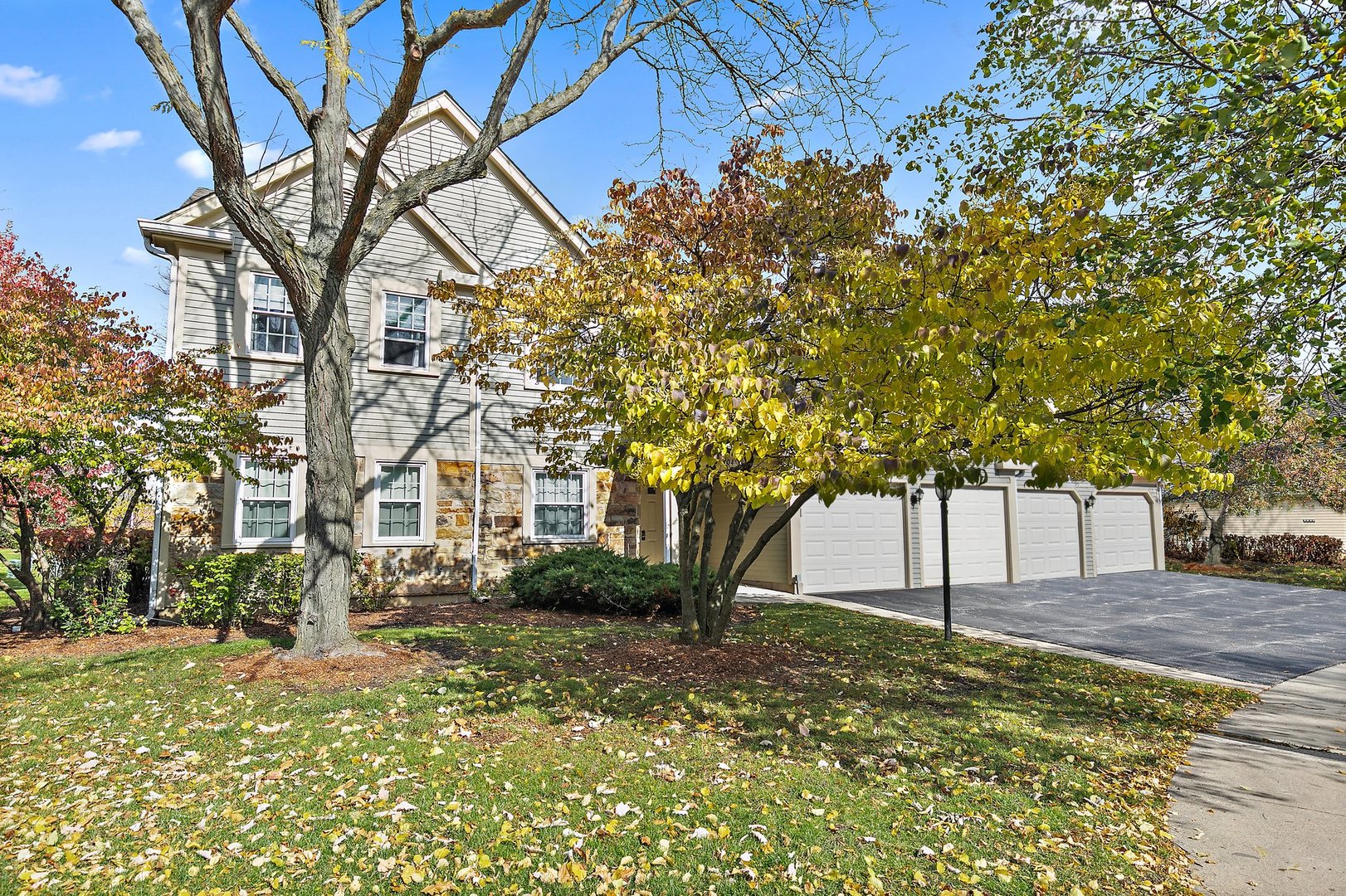This is an autumnal photograph of a substantial suburban house, likely marketed by a realtor. The house, a two-story structure with a potential attic room featuring expansive windows, showcases a mix of architectural elements including a lower brick facade and upper gray siding. Prominent in the photo is an attached four-car garage, underlining the home's considerable size. The wide, circular driveway adds a touch of elegance and suggests affluence. The setting is enhanced by a variety of trees in various stages of fall foliage, including a prominent bare tree in the foreground surrounded by trees with yellow, red, and green leaves, as well as manicured green grass and bushes nearby. The photo is set against a light blue sky with scattered small white clouds, making for an aesthetically pleasing and picturesque scene.